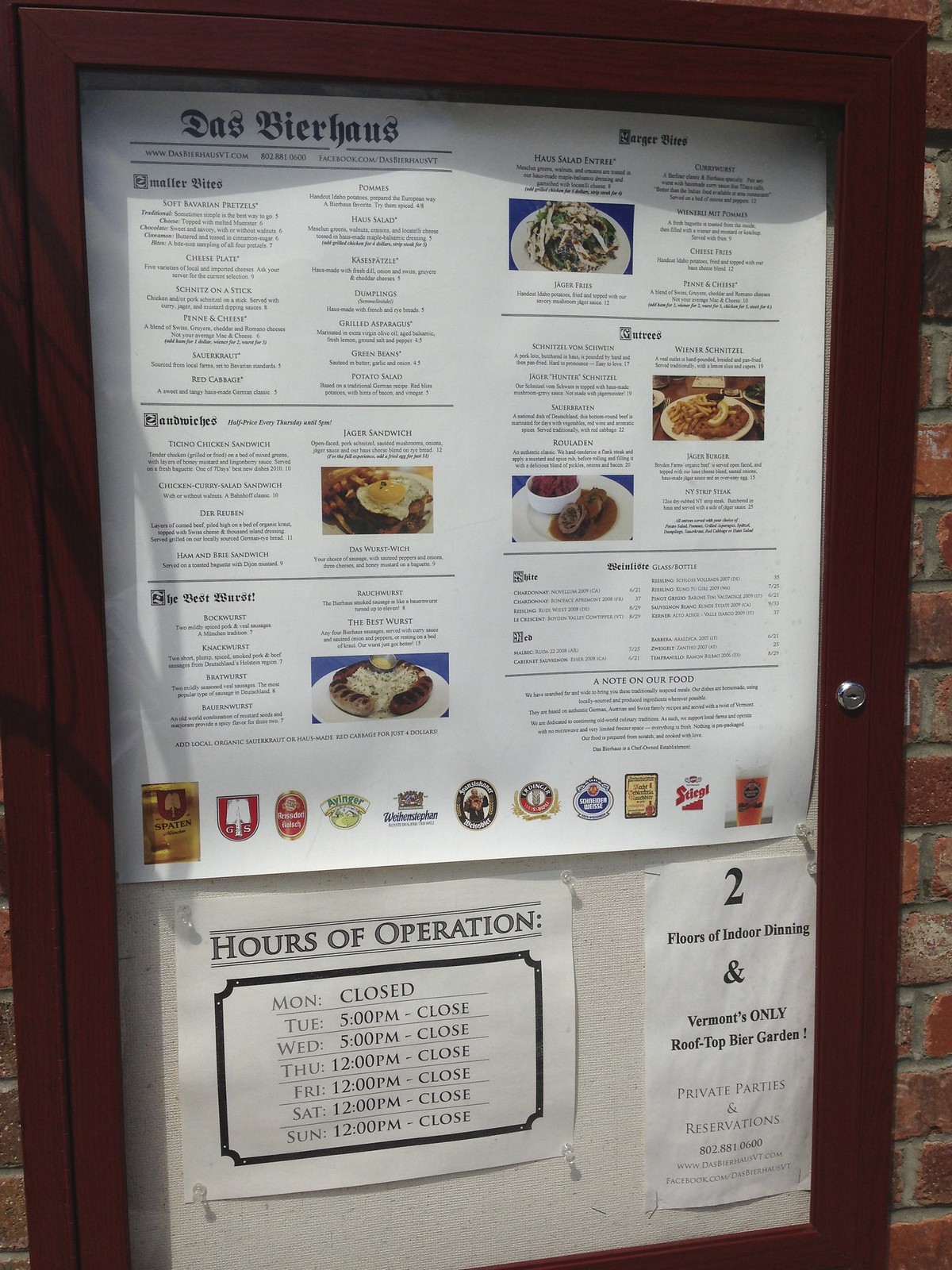In this photograph of a menu from a German restaurant, several printed papers are showcased within a brown wooden frame. The prominent piece of paper at the top is the main menu, titled "Das Bierhaus," indicating the restaurant's theme that highlights German cuisine and beer. The text on the menu is quite small, rendering it difficult to read most of the specific items and descriptions. However, it does include sections for "Smaller Bites," "Sandwiches," "The Best Wurst," "Burger Bites," "Entrées," and more. There are a few photographs accompanying the menu, displaying different dishes offered at the restaurant. At the bottom of the main menu, there is a list featuring images of various beer brands available.

Beneath the main menu, a smaller piece of paper outlines the restaurant's hours of operation: Monday (closed), Tuesday and Wednesday (5 p.m. to close), and Thursday through Sunday (12 p.m. to close). On the right side of the frame, another piece of paper advertises the restaurant's unique features with the text "Two Floors of Indoor Dining" and "Vermont's Only Rooftop Beer Garden."